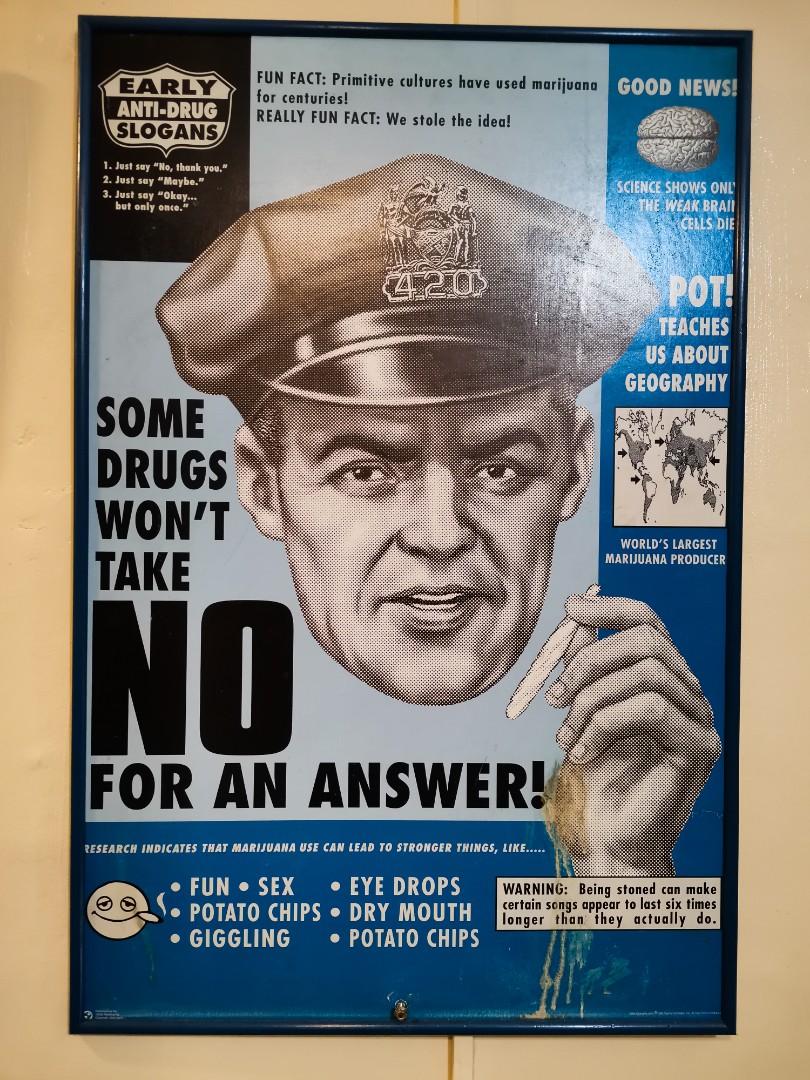This image features a large, humorous poster framed in black, prominently displaying an illustration of a stern-faced policeman at its center. The policeman, dressed in uniform with a cap labeled "420," holds a joint in his hand. Surrounding him is an array of whimsical and satirical anti-drug messages. In the top left corner, a shield reads "Early Anti-Drug Slogans," accompanied by numbered slogans such as "Just say no, thank you," "Just say maybe," and "Just say okay, but only some."

The top middle section includes quirky fun facts, noting "Primitive cultures have used marijuana for centuries," cheekily adding, "We stole the idea." The top right bears a brain with the text "Good news, science shows only the weak brain cells die." Below, a bold "POT!" declares it teaches geography, with an illustration of the world's largest marijuana producer.

Next to the policeman's face, a caption states, "Some drugs won't take no for an answer." An emoji with a joint in its mouth sits at the bottom left, alongside bullet points listing effects like fun, sex, potato chips, giggling, eye drops, and dry mouth. A warning at the bottom highlights, "Being stoned can make certain songs appear to last six times longer than they actually do." The overall blue-toned color scheme enhances the comedic yet thought-provoking nature of the poster, parodying the anti-drug messaging of the past.